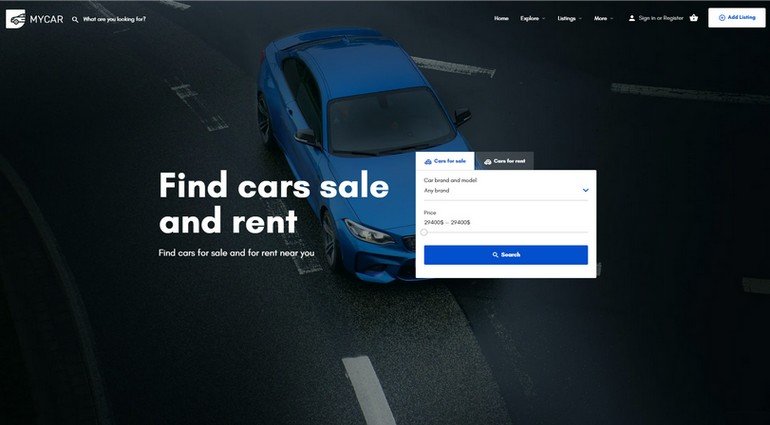The image is a screenshot from a website displayed in landscape orientation. The background is a dark photograph of an asphalt road with white striping, viewed from an aerial perspective. Dominating the foreground is a top-down view of a blue sedan positioned slightly off-center. The overall image appears somewhat ambiguous, leaving uncertainty as to whether it is a heavily modified photograph or an illustration.

In the upper left corner of the screen, there is a squarish white logo featuring a side view of the front end of a car. Next to the logo, the company's name "MY CAR NYC" is displayed in all uppercase letters. Adjacent to this logo is a small search bar. 

In the upper right corner, there are very small and hard-to-read menu options, including "Home" and "Sign In," with the rest being too tiny to identify clearly.

Superimposed over the photographic background, large white letters boldly proclaim "FIND CARS SALE AND RENT," despite the slight grammatical error. Beneath this prominent text, smaller white letters offer a grammatically correct message: "Find cars for sale and for rent near you."

Below this text lies a white rectangle containing two tabs, one selected in white and the other inactive in black, though the tab labels are undisclosed. There is also a dropdown menu likely intended for selecting car brands, and another dropdown for price range with an accompanying slider bar to adjust the desired price range.

At the bottom of this rectangle, a long blue search button is displayed, featuring the word "Search" and a magnifying glass icon, both rendered in white.